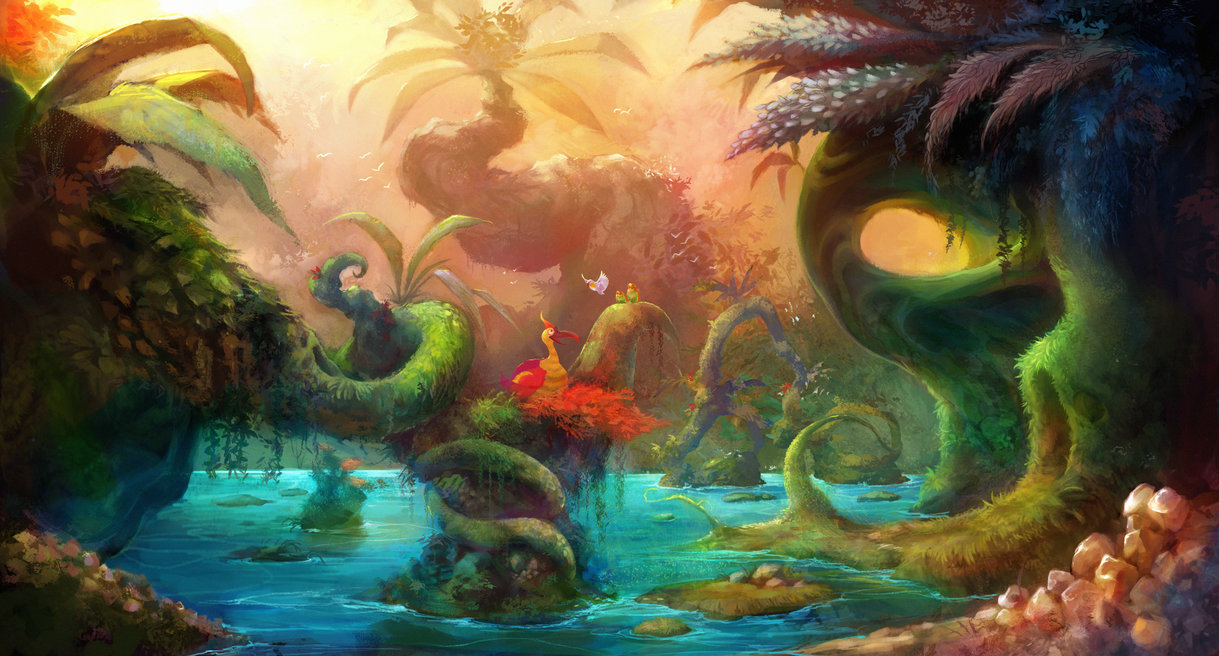The image is a colorful and fantastical scene of a mystical lagoon or pond, possibly a painting or computer-generated artwork. In the center, there is a bright blue pool of water, from which a peculiar V-shaped tree stump emerges, adorned with spiraling green vines. A vibrant yellow bird with red wings, a long red lacy feathered tail, and a red beak perches gracefully on this tree stump. Surrounding the lagoon, the landscape features large green plants with spiny leaves on the right, and a variety of green, yellow, and red foliage on the left, some of which overhang into the water. In the background, towering trees with flower petals and a palm-like peak curve sharply, casting shadows that blend into a yellow-hued sky reminiscent of a sunset. A small cave-like opening and a shoreline scattered with round, smooth rocks add to the scene's mystical ambiance.